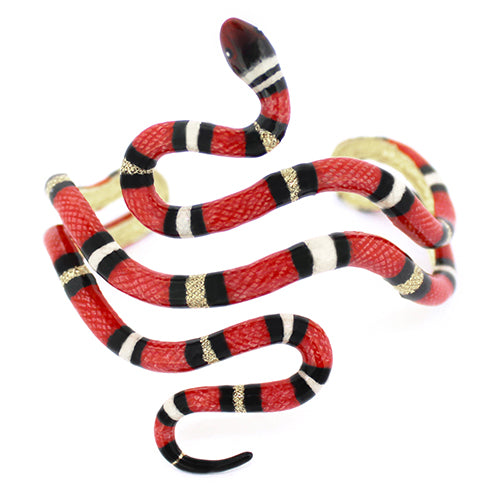The image features a highly detailed, artificial snake that curls back and forth against a plain white background. This painted snake, designed to resemble a stylish wrist bangle or bracelet, displays an elaborate pattern of alternating colors. The tip of its red head is situated at the top of the image, adorned with small white eyes encircled by black rings. Following the head, the body showcases a repetitive sequence of stripes: black, white, black, red, black, yellow with black dots, black, red, black, solid white, black, red, and so forth. The underside of its belly is a light yellow hue. The snake's coiled form, with a series of S-shaped curves, enhances its decorative appeal, making it an eye-catching accessory.